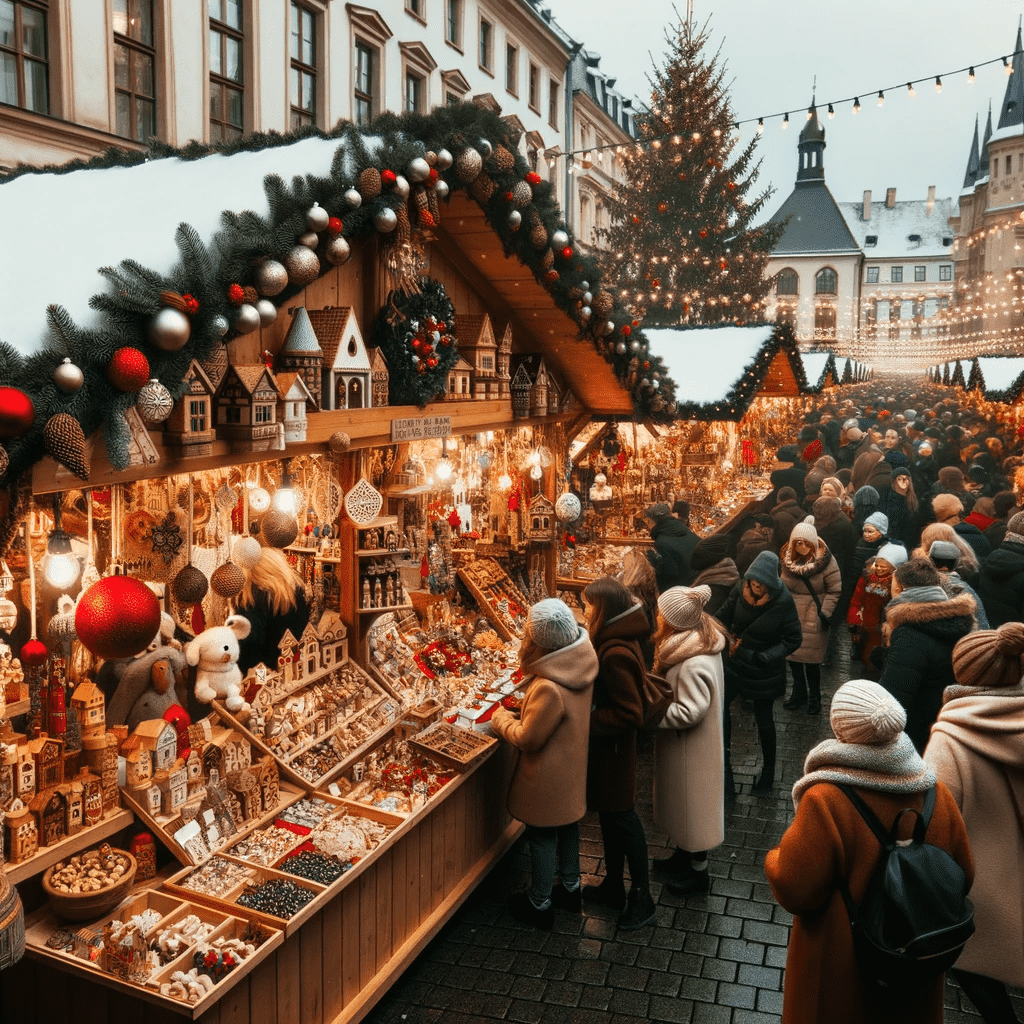The photograph captures a vibrant and bustling outdoor Christmas market set in a picturesque Bavarian town. Hundreds of people, dressed warmly in winter attire with toboggans, long overcoats, and scarves, wander through the market with a festive spirit. The scene is adorned with numerous kiosks decorated with Christmas ornaments, greenery, and lights, selling a variety of crafts including nutcrackers, small decorative houses, and other holiday trinkets. The market stalls are arranged on both sides of the street, creating a lively alleyway filled with holiday shoppers. The background reveals charming three and four-story buildings, with one distinctly featuring a steeple, contributing to the old-world charm of the setting. A large Christmas tree stands prominently lit with large white lights. Snow blankets the roofs, adding to the wintry ambiance, and the cobblestone streets reflect a slight wetness, enhancing the enchanting, festive atmosphere of this European Christmas market.